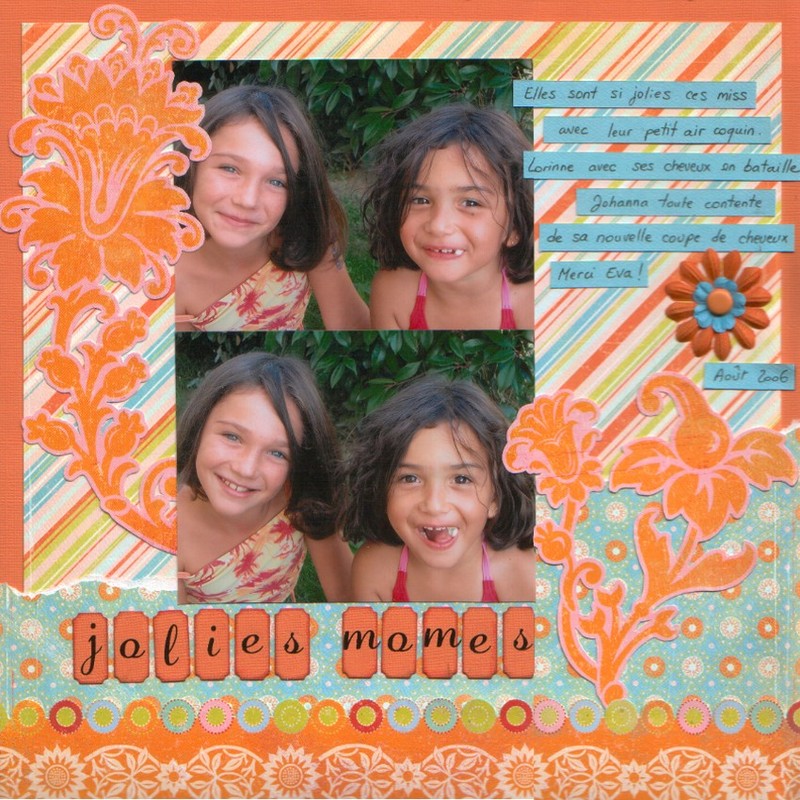This image depicts a vibrant scrapbook page with a coral orange background adorned with diagonal stripes in shades of orange, green, and light pink. In the left-hand corner, two cutout flowers, colored in orange and pink, accent the page. The center features two color photographs, one above the other, showcasing two girls with light skin and short brown hair. In the top photograph, the girl on the left, with thin, short brown hair, wears a yellow dress adorned with pink palm trees and smiles with her mouth closed. The girl on the right, sporting wavy or curly, messy short brown hair and a pink halter top, smiles with her mouth slightly open. In the bottom photograph, the same girls switch their expressions: the left girl smiles with her mouth slightly open, while the right girl laughs with her mouth wide open. Both photographs are surrounded by a fancy frame of flowery patterns in shades of pink and orange. Scattered text and several blue strips of paper with handwritten notes embellish the right side of the page. At the bottom, rectangular orange labels bear the words "Jollies" and "Mommies," celebrating the friendship between these two young girls.